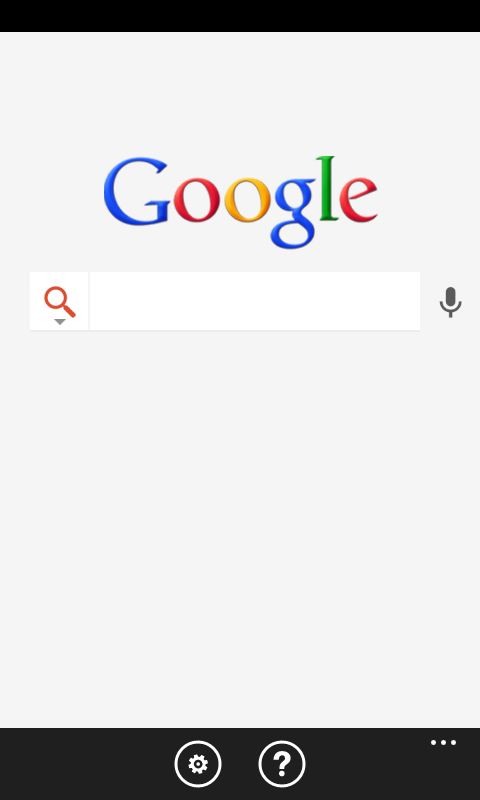This image depicts a screenshot from a smartphone displaying a Google search page. The upper and lower borders of the screen are solid black. The main body of the screen has a very light gray background. Prominently located in the top third of the screen is the colorful Google logo. Below the logo is a search box that includes a gray search icon on the left side and a drop-down arrow, with a gray microphone icon on the right side of the search box. At the bottom of the screen, there is a black border featuring three icons: a settings icon, a question mark icon, and three horizontal dots. The screenshot captures the familiar "I'm Feeling Lucky" Google homepage interface, recognizable from traditional browsers, but viewed here on a smartphone.